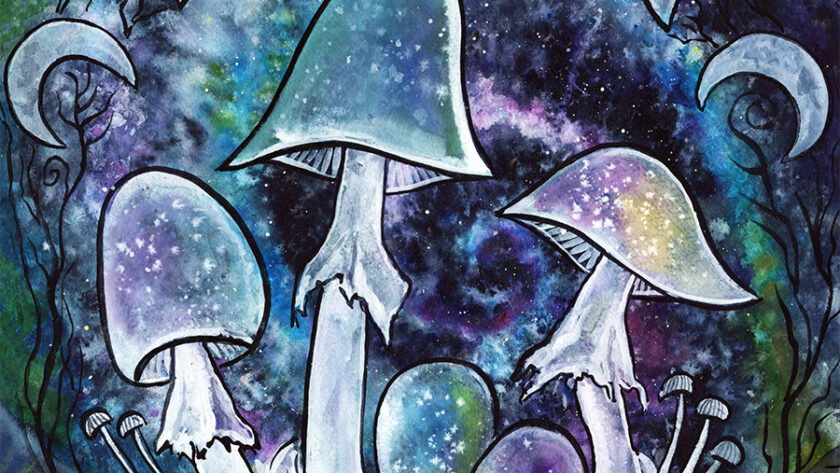The image is a large oil painting featuring a psychedelic scene with a dark background dominated by deep purples, dark blues, and blacks, peppered with green highlights. At the center, three large, white mushrooms stand prominently, each adorned with unique logos and symbols. Surrounding these main mushrooms are several smaller ones, adding to the intricate detail. The background appears to have a galaxy theme, with numerous stars, crescent moons on both the left and right sides, and a mystical, ethereal feel. The use of varied colors and shading throughout the painting, along with its dreamy and surreal elements, gives it a captivating and otherworldly quality.